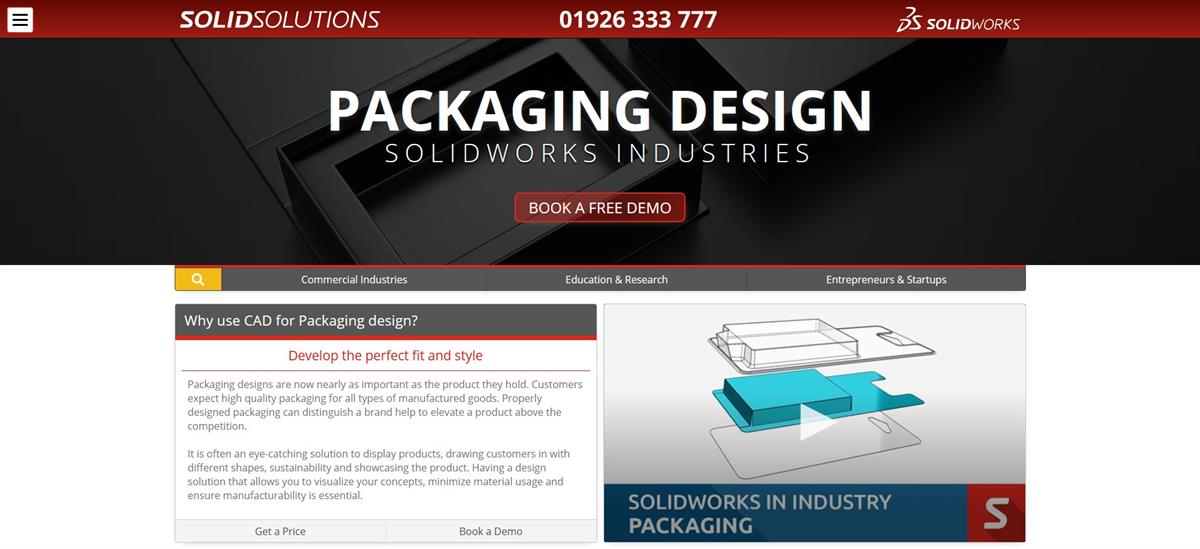The image displays a screenshot from a website with a structured and professional design. 

At the top, there is a deep burgundy or crimson banner. On the left side of this banner, a small white square contains three equally spaced horizontal black lines, resembling a menu icon. Adjacent to this, the text "SOLID SOLUTIONS" is prominently displayed in bold, capital letters followed by a phone number, "01926333777," and the phrase "Solid Works."

Below this header, the background transitions to black, showcasing various products depicted as squares or boxes. Superimposed on this background, the white text reads: "Packaging Design, Solid Work Industries." Additionally, a call-to-action button with the text "BOOK A FREE DEMO" in white, capital letters encourages viewer interaction.

Further down, a white background is introduced, topped with a gray banner. This banner includes a small marigold yellow square with a white magnifying glass icon within it. The gray banner also lists several links in white text: "Commercial Industries," "Education and Research," and "Entrepreneurs and Startups."

Continuing down, there is a gray-topped box labeled "Why Use C8A for Packaging Design." A red line divides the section, beneath which the phrase "Develop the Perfect Fit and Style" is highlighted. This section also contains a brief paragraph with options to "Get a Price" or "Book a Demo."

On the right side, the text "Solid Works in Industry Packaging" is positioned alongside a square with an "S" inside, encapsulating the theme of the website.